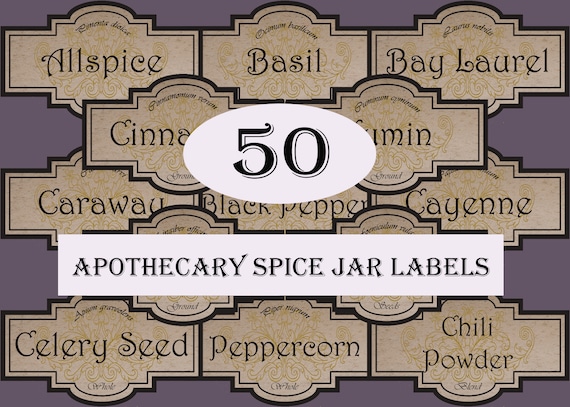This horizontally aligned rectangular image features a solid gray background, but most of it is covered by various spice jar labels. Prominently in the center, there is a white oval displaying the number "50" in black. Directly below this oval, a white rectangle contains the text "APOTHECARY SPICE JAR LABELS" in black, all capital letters. The backdrop consists of tan, shaded shapes each labeled with the name of a spice in black font. Starting from the upper left and moving across, the visible labels read "Allspice," "Basil," "Bay Laurel," "Cinnamon" (partially obscured showing "CINNA"), and "Cumin" (partially covered by the oval showing "UMIN"). In the center row, the labels include "Caraway," "Black Pepper," and "Cayenne," with two additional labels entirely obscured by the white rectangle. Finally, the bottom row shows "Celery Seed," "Peppercorn," and "Chili Powder." The overall image is clear and bright, ensuring the text is easy to read.